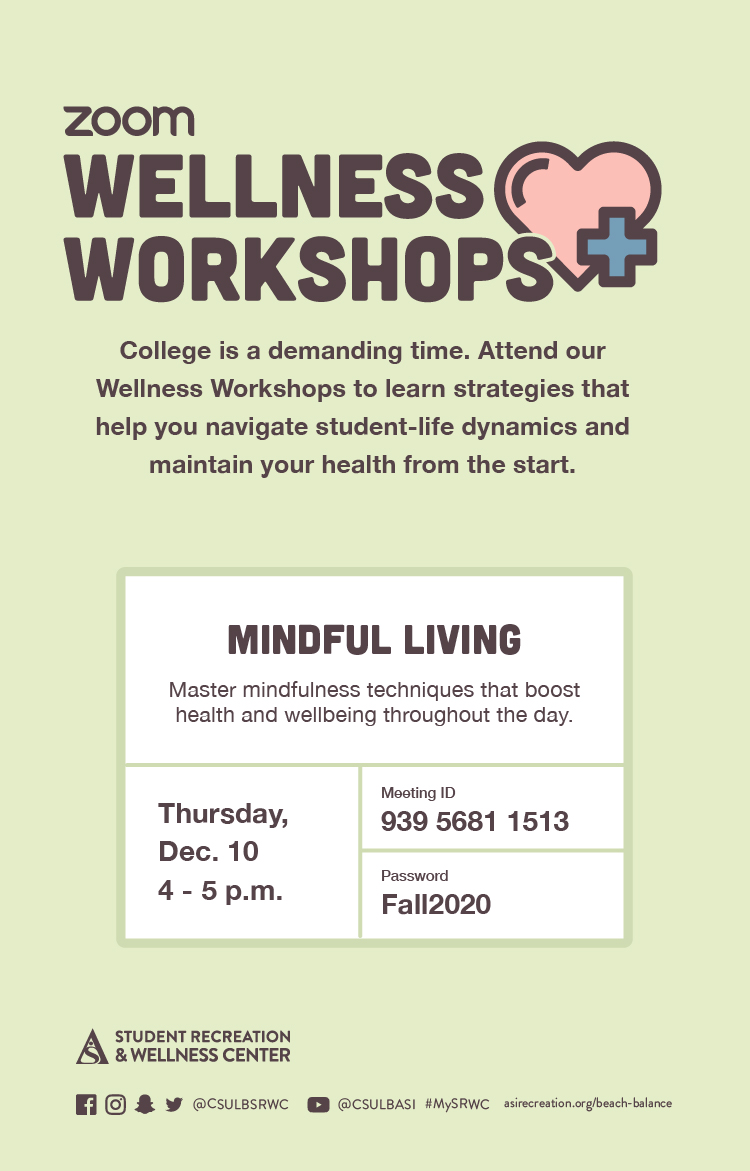The advertisement screenshot, displayed in portrait orientation against a gray background, is approximately twice as tall as it is wide. At the top of the ad, the word "Zoom" is prominently featured. Below it, in larger black font, the title "Wellness Workshops" is displayed, accompanied by a heart-shaped graphic with a black border, a pink interior, and a blue plus sign on its bottom-right corner.

The caption beneath the heart graphic reads, "College is a demanding time. Attend our wellness workshops to learn strategies to help you navigate student life dynamics and maintain your health from the start."

A green-bordered box encloses the lower half of the advertisement. The top section of this box spans horizontally and occupies half of the page, with the heading "Mindful Living" and the description, "Master mindfulness techniques that boost health and well-being throughout the day."

The bottom half of the green-bordered box is divided into three sections. The left half contains a date and time: "Thursday, December 10, 4 to 5 p.m." Adjacent to it is a horizontal box featuring a meeting ID. Below this, another box provides the meeting password: "fall 2020."

Near the bottom of the advertisement is an icon resembling a triangle with the text "Student Recreation and Wellness Center." Below, social media icons for Facebook, Instagram, Snapchat, and Twitter are displayed, followed by additional informational text.